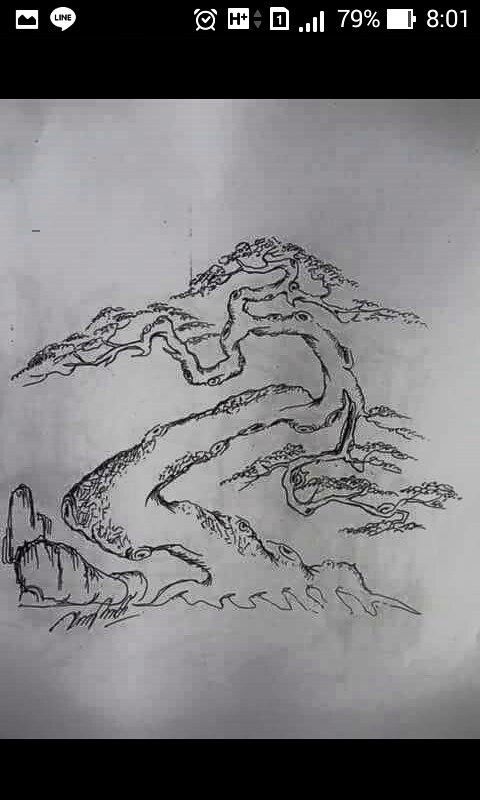Here is a cleaned-up and detailed caption for the image:

---

This black-and-white illustration captures a hand-drawn tree intricately rooted into the ground. The tree's trunk twists and turns to the left, then snakes back to the right, finally curving leftward again, creating a dynamic and flowing form. The branches display a whimsical, swirling pattern, adorned with bits of foliage. The trunk and branches are detailed with knots that resemble eyes or open mouths, inviting viewers to find hidden images within the tree's form. To the left of the tree, a cluster of sketched boulders adds a sense of grounding to the scene. The artist's signature is delicately inscribed near the boulders on the left, completing the piece.

---

This description aims to provide a vivid and comprehensive portrayal of the image, allowing a reader to visualize it without seeing it.